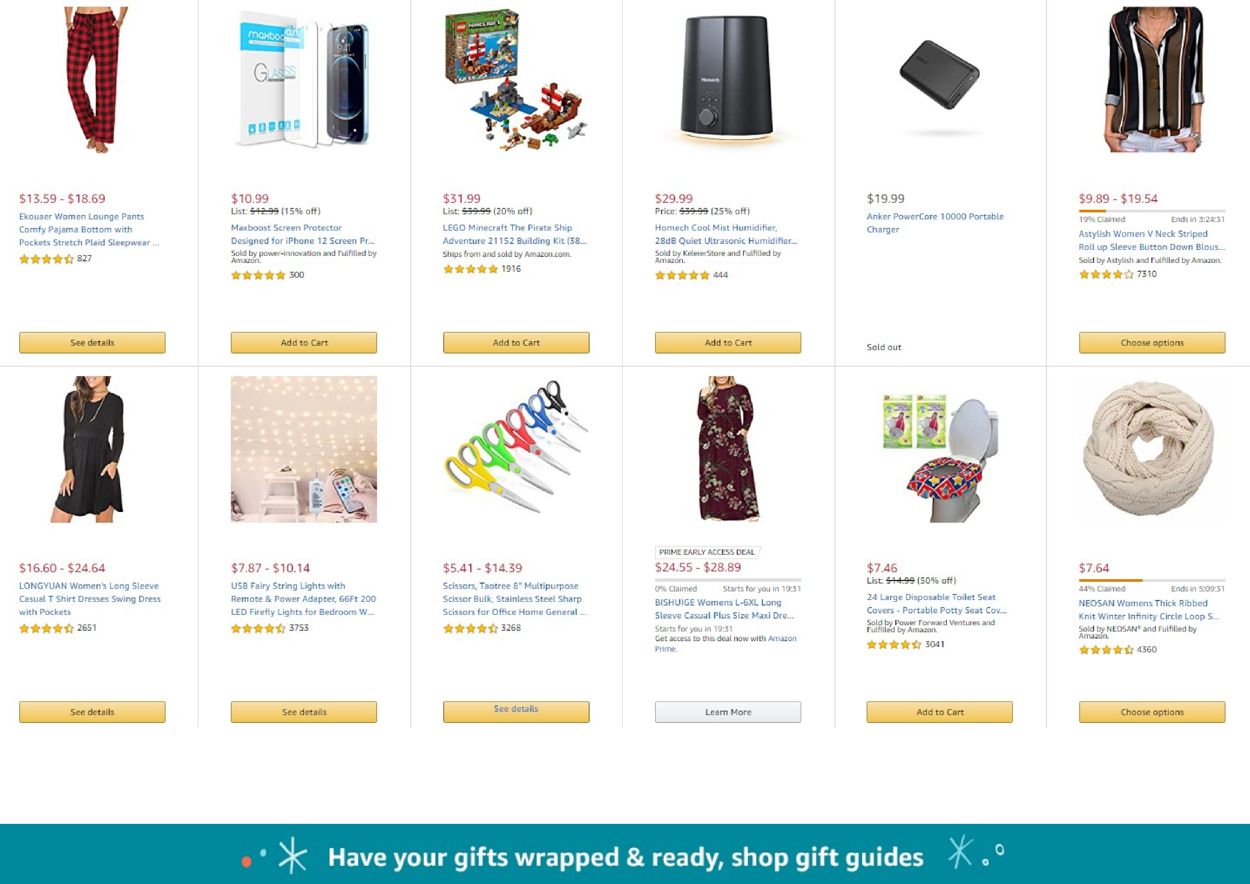This page displays an Amazon search result for items on sale, arranged in two rows with six items each, moving from left to right.

In the top left corner, there is an item priced between $13.59 and $18.69. It features Women's Lounge Pants described as "Comfy Pajama Bottom with Pockets, Scratch Plaid Sleepwear," rated 4 stars based on 927 ratings.

To its immediate right, another item is priced at $10.99 with a listed price of $12.99, reflecting a 15% discount. It is the "Max Boost Screen Protectors" designed specifically for iPhone 12 screens.

Next to it, an item priced at $31.99 (originally $35.99, showing a 20% discount) is the "Lego Minecraft, The Pirate Ship Adventure 21152 Building Kit."

Following that, another item is priced at $29.99.

Additional details or descriptions for the remaining items on the rows are not provided.